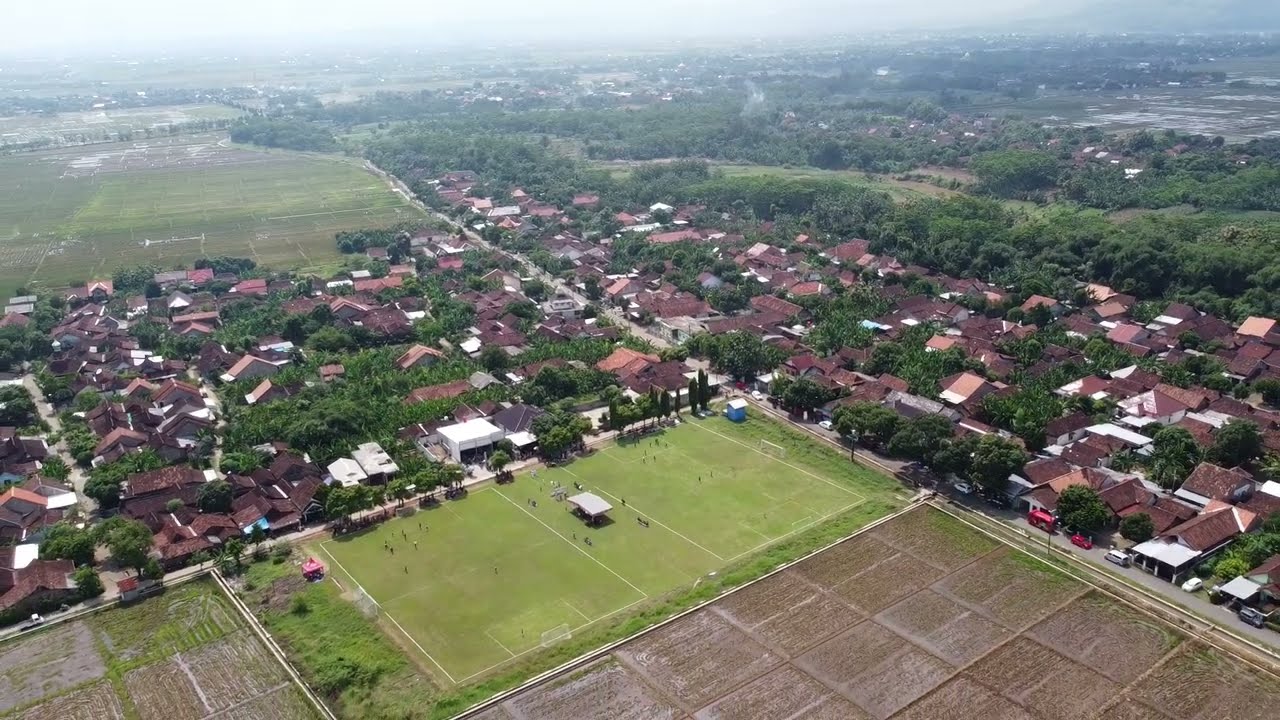This is a detailed aerial view of a neighborhood, likely captured from a small airplane or a drone, several hundred feet above the ground. The photograph is angled, providing a sweeping perspective of the landscape. At the top of the image, the horizon fades into a hazy atmosphere. 

In the center of the photograph, there are two adjacent soccer fields with clearly marked outlines. Between them is a tent-like structure, suggesting a celebration or festivity taking place. People are visible in this area, enhancing the sense of activity. 

Towards the bottom of the image, several farming fields are prominently displayed. These fields are mostly brown, indicating they might be either tilled or lying fallow. 

On the left side of the photograph, a cluster of houses with brown and red tile roofs is surrounded by numerous trees. These houses are closely packed, forming a distinct neighborhood. A diagonal, two-lane road runs from the center-right of the soccer fields toward the upper right corner of the image, acting as a boundary between different sections of the neighborhood. 

On the right side of the road, another dense collection of houses mirrors the left side, with more trees interspersed among them. Beyond these houses, the landscape shifts to a mixture of trees and more agricultural fields, which appear slightly more hilly in the distance. The roads connecting these sections weave through the communities, linking various parts of the neighborhood.